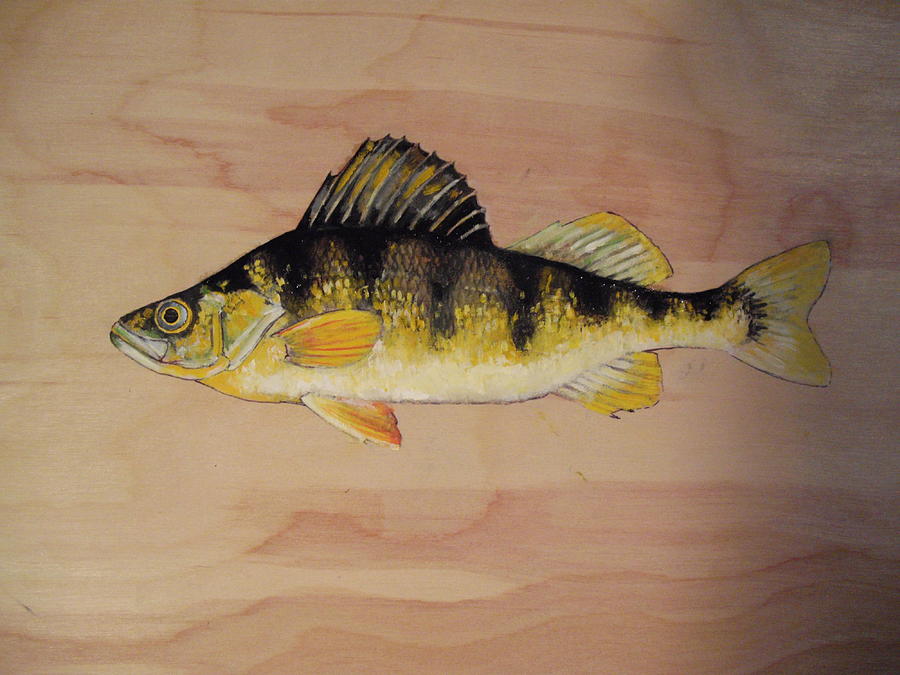This square image features a detailed painting of a fish on a light wooden surface, possibly a tabletop. The light wood has horizontal, slightly curved grain patterns. The fish, oriented with its head to the left and mouth closed, has a striking coloration: the top part of its body is black transitioning into gold, with the bottom part being a mix of pale yellow and white. The fish's fins are primarily gold, with the top fin displaying a blend of black and gold stripes. The tail fin is gold tinged with white. The fish's large eye has a black center outlined in gold, encircled by a brown ring and another gold border. The painting appears to be acrylic, as it rests cleanly atop the wood, suggesting it hasn't soaked in. The fish also features finely detailed black stripes that point towards the belly and fade out, adding to the intricate design. Elements of yellow, brown, and white scales add to the rich texture of the fish's body, making it an eye-catching centerpiece on the wooden surface. Shadows to the right of the fish indicate a light source from the left, adding depth to the image.